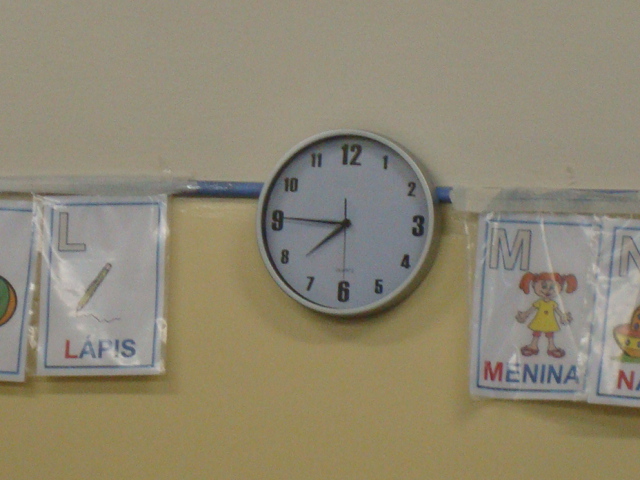This photograph appears to have been taken inside an elementary school classroom, featuring a beige wall with a darker beige section below a blue horizontal trim. In the center of the image, a simple wall clock displays the time as a quarter till eight. The clock is encased in a plain beige or grayish silver housing with a white face and black hands, including a second hand. The numerals 12, 3, 6, and 9 are prominently larger than the other numbers. Surrounding the clock are small alphabet posters laminated in clear plastic sheet protectors and taped to a gray conduit supplying power to the clock. On the left side, we see the letter "L" with an image of a pencil labeled "lapis." On the right side is the letter "M" with an illustration of a red-haired girl labeled "menina." Additionally, part of the letter "N" is visible with what seems to be an image resembling a bowl. The scene is well-lit with reflections visible on the plastic laminate.